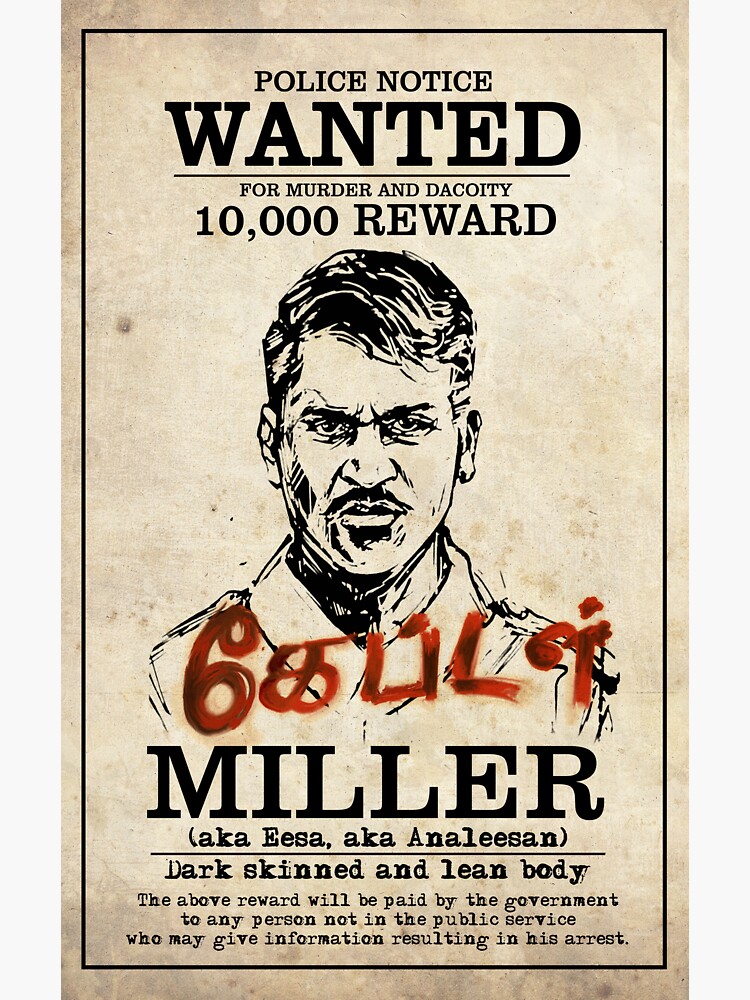This is an old-fashioned wanted poster featuring a black and white line drawing of a dark-skinned, lean man with short black hair, furrowed eyes, and a small dark mustache. At the top, in white trim, it reads "Police Notice" followed by the underlined word "WANTED." The man, identified as Miller, aka Essa, aka Annalisa, is wanted for murder and decoity, with a reward of $10,000 offered by the government to any person not in public service who provides information leading to his arrest. The drawing shows the man wearing a white jacket, with a scowling expression and crinkled nose, enhancing his menacing appearance. Written across the poster in red graffiti, partially obscuring Miller's photo, are unknown characters that do not appear to be in English.